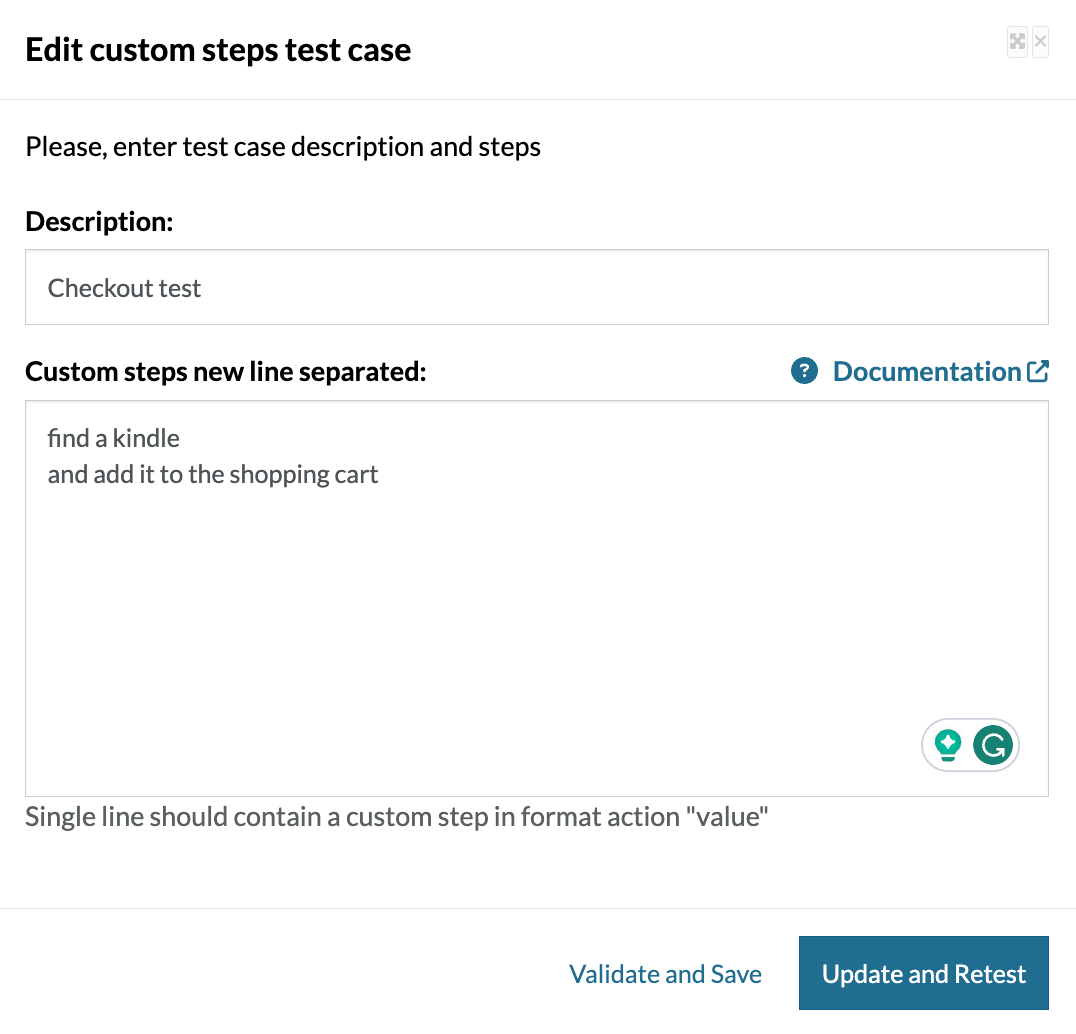The screenshot depicts a section of an unnamed website where users can edit custom steps, presumably for creating or managing test cases. The interface includes two primary input fields: the first is a single-line box for the test case description, and the second is a larger, multi-line box for detailing the custom steps, with each step separated by new lines. In the description field, there is an entry that reads, "check out test." The custom steps field contains a single step: "find a Kindle and add it to the shopping cart." 

To the right of the input fields, there is a button labeled "Documentation" marked with a question mark inside a circled icon, presumably offering help or guidance. At the bottom of this section, there is an instructive note that reads, "Single line should contain a custom step in format, action 'value'." The interface concludes with two actionable buttons— "Validate and Save" and "Update and Retest."